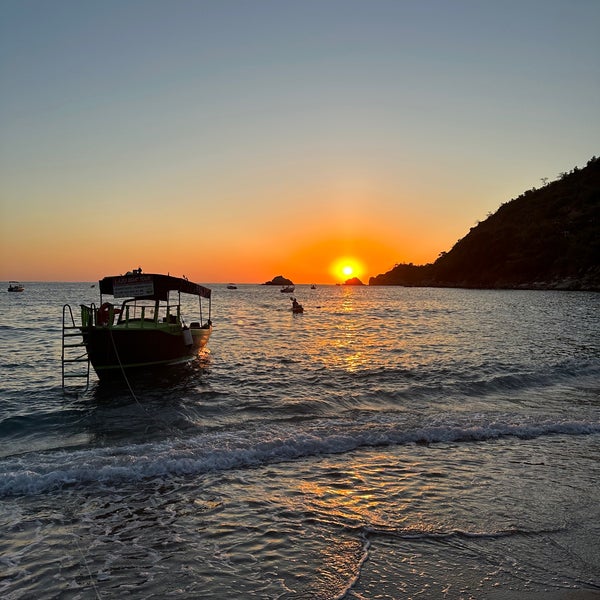The photograph captures a serene waterfront scene at sunset, showcasing a small boat with a roof anchored close to a shore, facing the camera. The boat features a ladder on its left side, extending down into the water of what appears to be a lake, bay, or part of the ocean. The waves are gently choppy, creating a light surf near the shore. In the backdrop, the bright yellow sun is setting, casting an orange aura in the gradient blue sky, with a white circular center. To the right, a hilly and mountainous landscape adorned with forest stands in contrast to some visible rocks near the water. The beautifully composed image reflects a tranquil moment with the sun barely above the ocean's rocks, enhancing the picturesque and calm atmosphere.